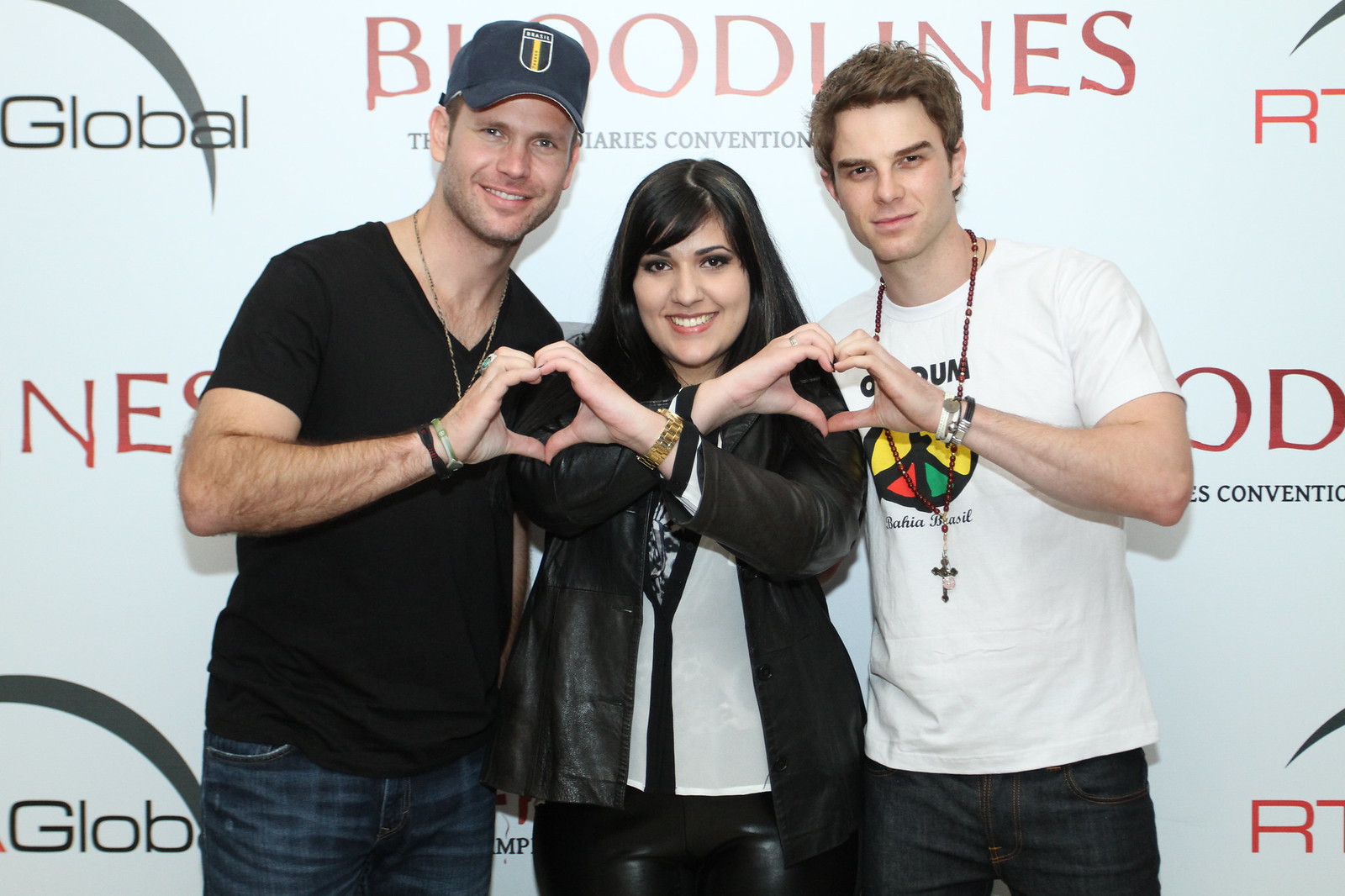This detailed, full-color photograph captures three individuals posing indoors at the Bloodlines: The Vampire Diaries Convention. The trio stands in front of a repeating white banner that partially displays the convention's name along with a company logo. Their arms are interlocked, collectively forming heart shapes with their hands – a gesture popular in fan photos.

On the left is a taller man donning a black baseball cap, a black t-shirt, a necklace, a blue and black wristband, and denim jeans. On the right stands another man wearing blue jeans, a white t-shirt emblazoned with "Brazil," and a cross necklace; he appears to be grimacing slightly. Centered between the two men is a shorter woman with dark brown hair. She’s smiling brightly at the camera, dressed in a black leather jacket, black leather pants, and a white undershirt with a print design.

The men are actors from The Vampire Diaries – Nathaniel Buzalik on the right and Matt Davis on the left – posing with a fan whose outfit and joyous demeanor add to the friendly atmosphere of the photograph.